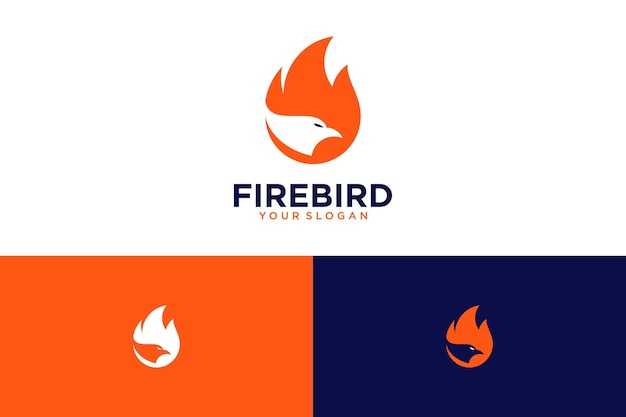The image, a PNG file with a predominantly white or translucent background, is approximately 6 to 7 inches wide by 5 inches tall. It features a central flame icon with three orange prongs, incorporating a white bird’s head in the negative space on the left side. Directly below this, in dark blue block letters, it reads "FIREBIRD," followed by the slogan "YOUR SLOGAN" in smaller orange block letters. The lower section of the image is divided into two equal blocks: on the left, an orange block with a white flame cutout that encloses a matching orange bird profile, and on the right, a dark blue block with an orange flame containing a blue version of the bird’s profile. The consistent use of the flame and bird motif suggests various design options for a logo, emphasizing a cohesive brand identity.